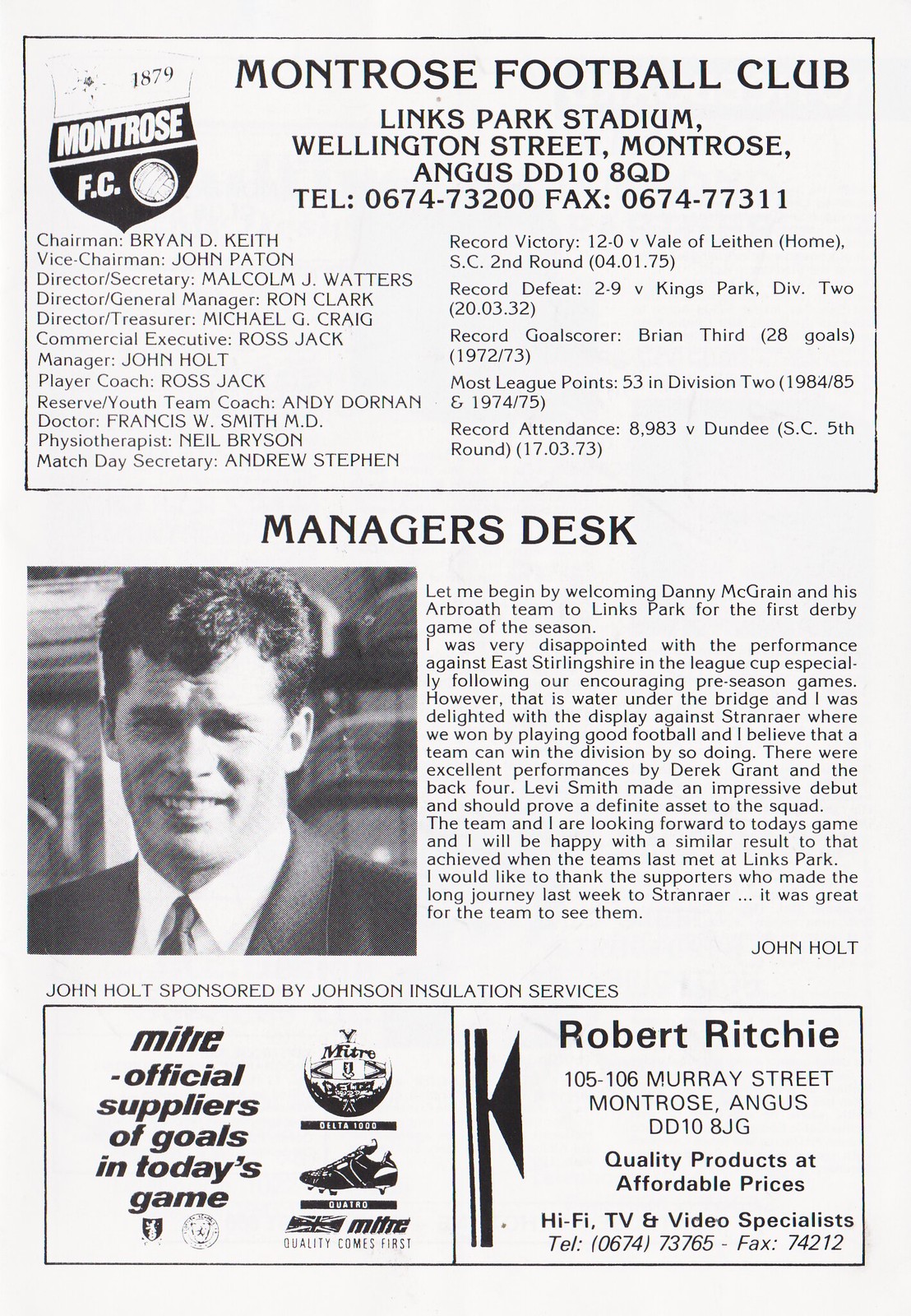The image appears to be a detailed black and white page from a publication, specifically a soccer flyer or a newspaper advertisement for the Montrose Football Club. At the top, a bold headline reads "Montrose Football Club" followed by the club's address: Links Park Stadium, Wellington Street, Montrose, Angus, DD10 8QD. Contact details include Telephone 0674-73200 and Fax 0674-77311. Prominently displayed is the club’s logo, a shield with the inscription "Montrose FC" and "Est. 1879." 

Alongside and below the logo, there's a comprehensive list of club officials including the Chairman, Vice Chairman, Directors, Secretary, Coaches, and medical staff. Detailed club history is also provided with notable records like a record victory of 12-0 against Vale of Leithen and a record defeat of 2-9 against Kings Park. 

In the middle of the page, under "Manager's Desk," there is a black and white photograph of the manager, John Holt, dressed formally in a suit and tie. The text above the photo serves as an editorial, where Holt welcomes Danny McGrain and his team to Links Park and reflects on a disappointing performance against East Sherlington in the Team League Cup, despite a promising preseason. The editorial is signed and sponsored by Johnson Insulation Services.

At the bottom of the page, there are advertisements for local businesses supporting the team, including Robert Ritchie, a hi-fi TV and video specialist located at 105-106 Murray Street, and Miltray, the official suppliers of goals for the day's game, featuring an image of a soccer cleat and ball. All text is in black on a white background, contributing to the classic and formal presentation of the page.